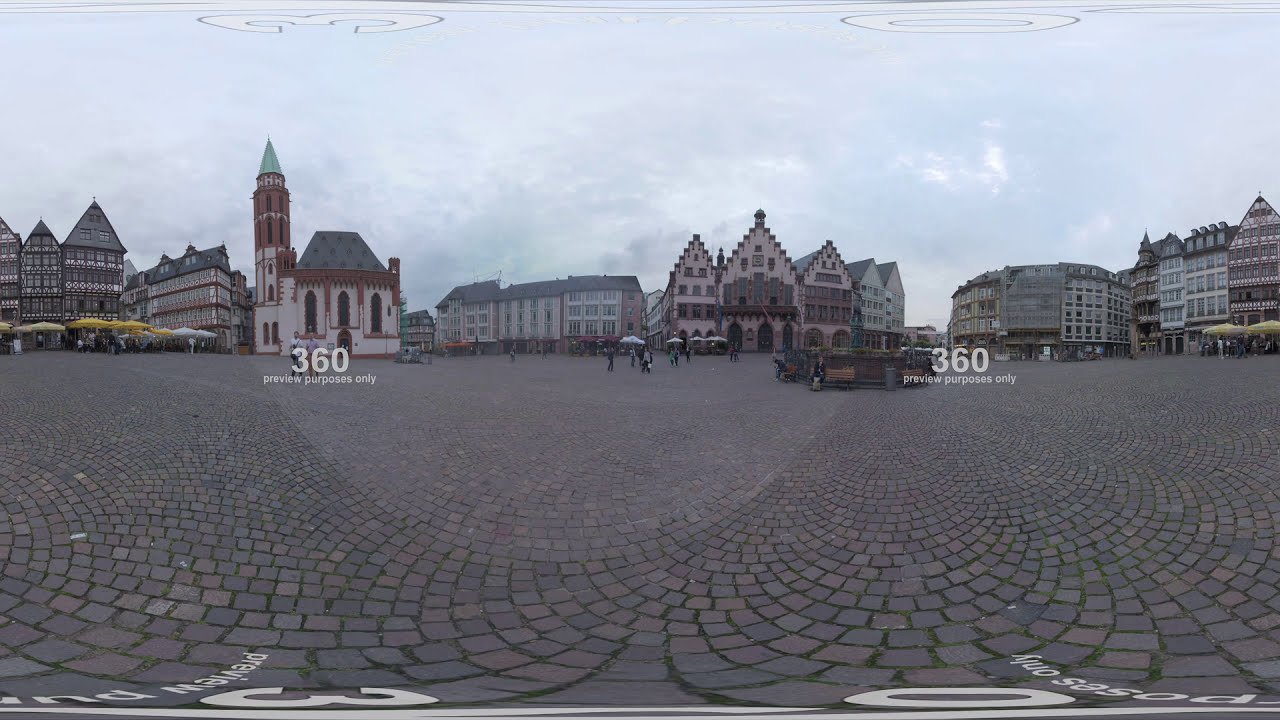The image depicts a large, gray-bricked courtyard situated in front of grand, palace-like buildings with distinct Old World architectural features, reminiscent of a European city, possibly resembling Amsterdam or an English or Dutch town. The buildings exhibit a mix of tan and copper colors with gray roofs and are evocative of medieval castles or structures from a fairytale, showcasing a unique architectural style. Crowds of people walk through the courtyard, some carrying white umbrellas, under a predominantly cloudy sky with glimpses of blue. The scene also includes several yellow and white awnings adorning the fronts of the buildings. In the image, “360 preview purposes only” is displayed in white text, indicating a panoramic view. On the left, there is a tall white house with a steeple, while the right side reveals a large three-sectioned building, alongside a row of tall, narrow houses, and a round building. The courtyard and its surroundings have an air of historical mystique, as if straight out of a legendary narrative.